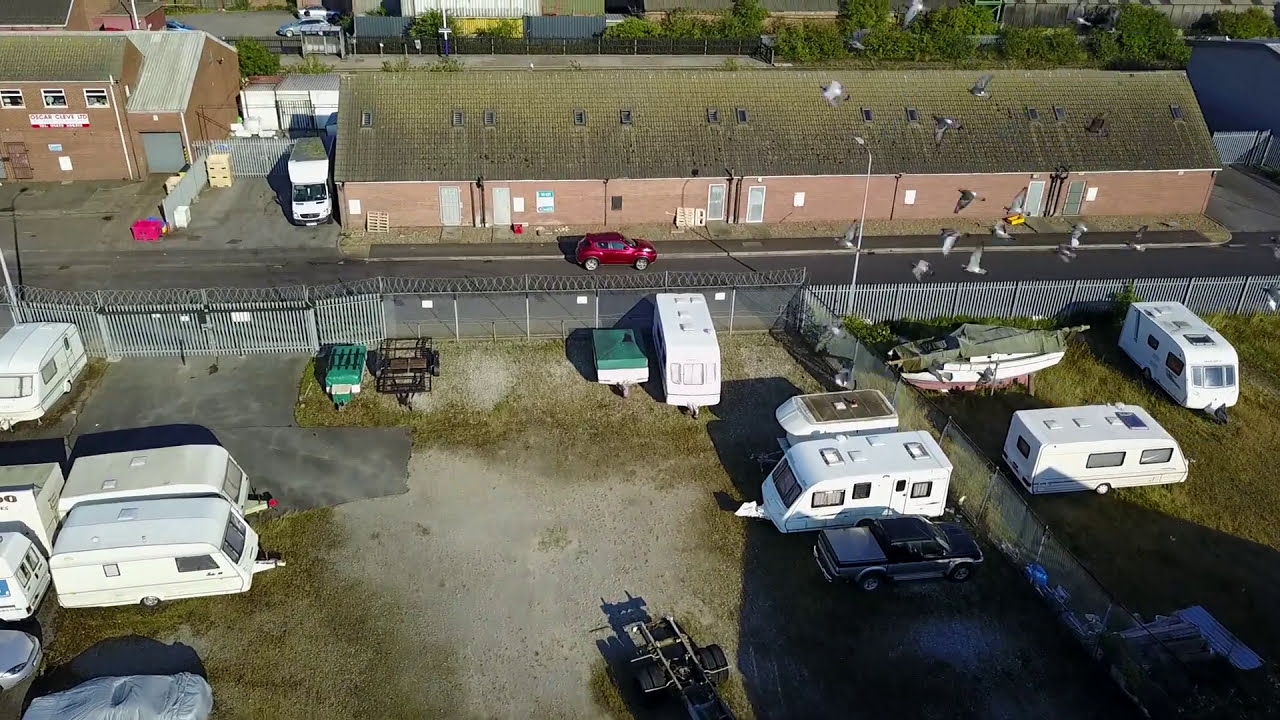This overhead shot captures a diverse urban scene divided by a small street running through the image. In the foreground, a fenced-off area is dominated by a collection of uniform, whitish RVs and a boat, suggesting either a city caravan park or an RV retailer. The area is secured by a metal fence topped with razor wire. Scattered around the enclosure are a few vehicles, including a truck, and various pieces of equipment. On the opposite side of the street, a red car is either parked or in motion. The background features a long, brick building that looks vaguely industrial, perhaps repurposed as cheap housing, with a moss-covered roof and flanked by trees. Additional buildings and driveways can be discerned behind it, along with parked trucks. The scene is bathed in sunlight, casting long shadows and capturing a few pigeons flying above the street, adding to the static yet detailed atmosphere of the image.